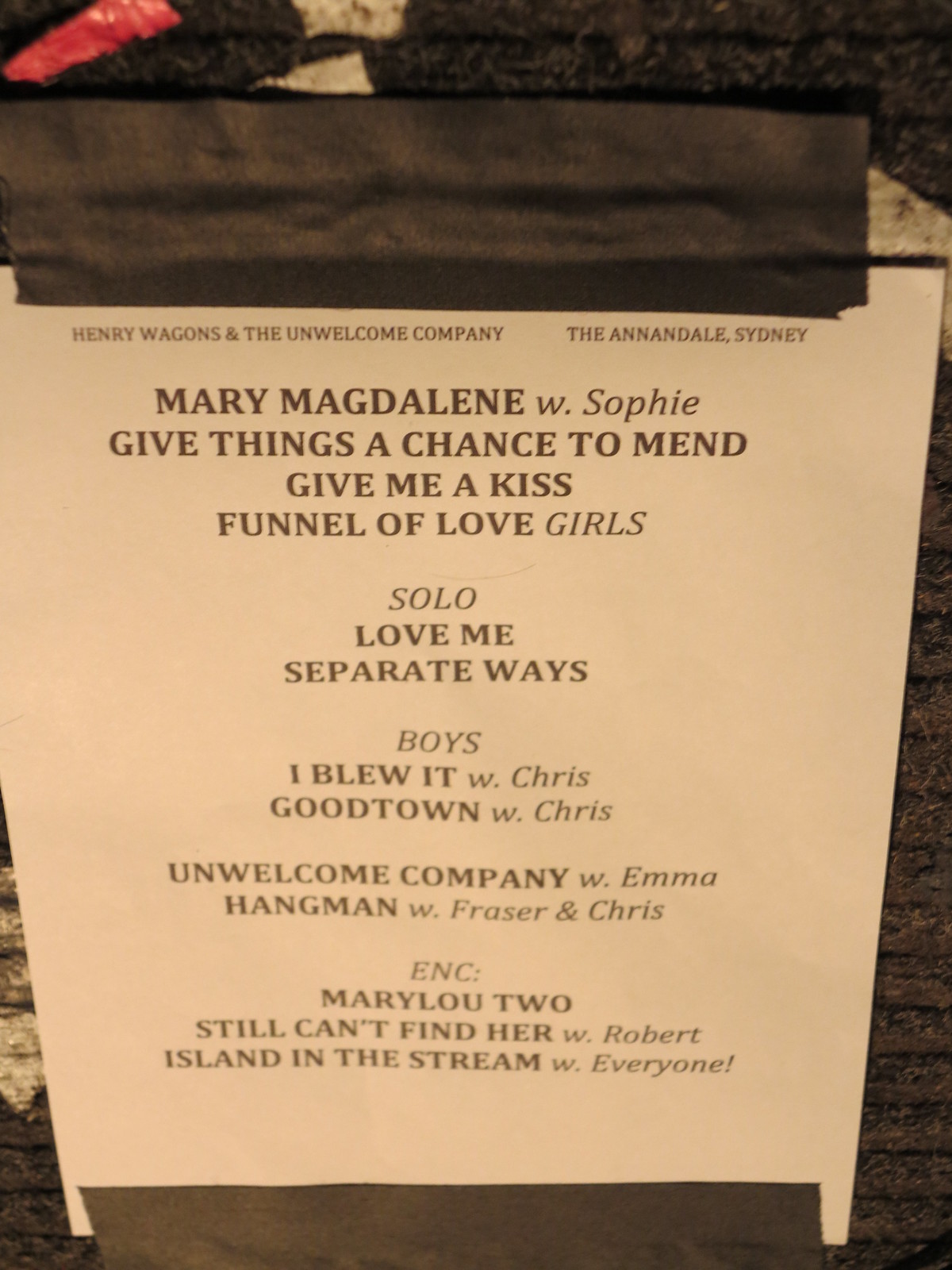The image depicts a black-and-white, sepia-toned flyer taped horizontally with black duct tape to a black, ridged, fabric-textured wall. This flyer serves as a program or schedule for an event headlined by Henry Wagons and the Unwelcome Company at the Annadale in Sydney. The top of the flyer, in small, all-caps text, reads "Henry Wagons and the Unwelcome Company" followed by "the Annadale, Sydney". The main body of the flyer lists various songs and performers in bold black font: "Mary Magdalene, W.Sophie," "Give Things a Chance to Mend," "Give Me a Kiss," "Funnel of Love, Girls," "Solo," "Love Me," "Separate Ways," "Boys," "I Blew It, W.Chris," "Good Town, W.Chris," "Unwelcome Company, W.Emma," and "Hang Man, W.Fraser and Chris." An additional mention includes "Encore: Mary Lou Too" and other shared performances like "Still Can't Find Her" and "Island in the Stream with Everyone." This detailed listing suggests a structured musical performance event.